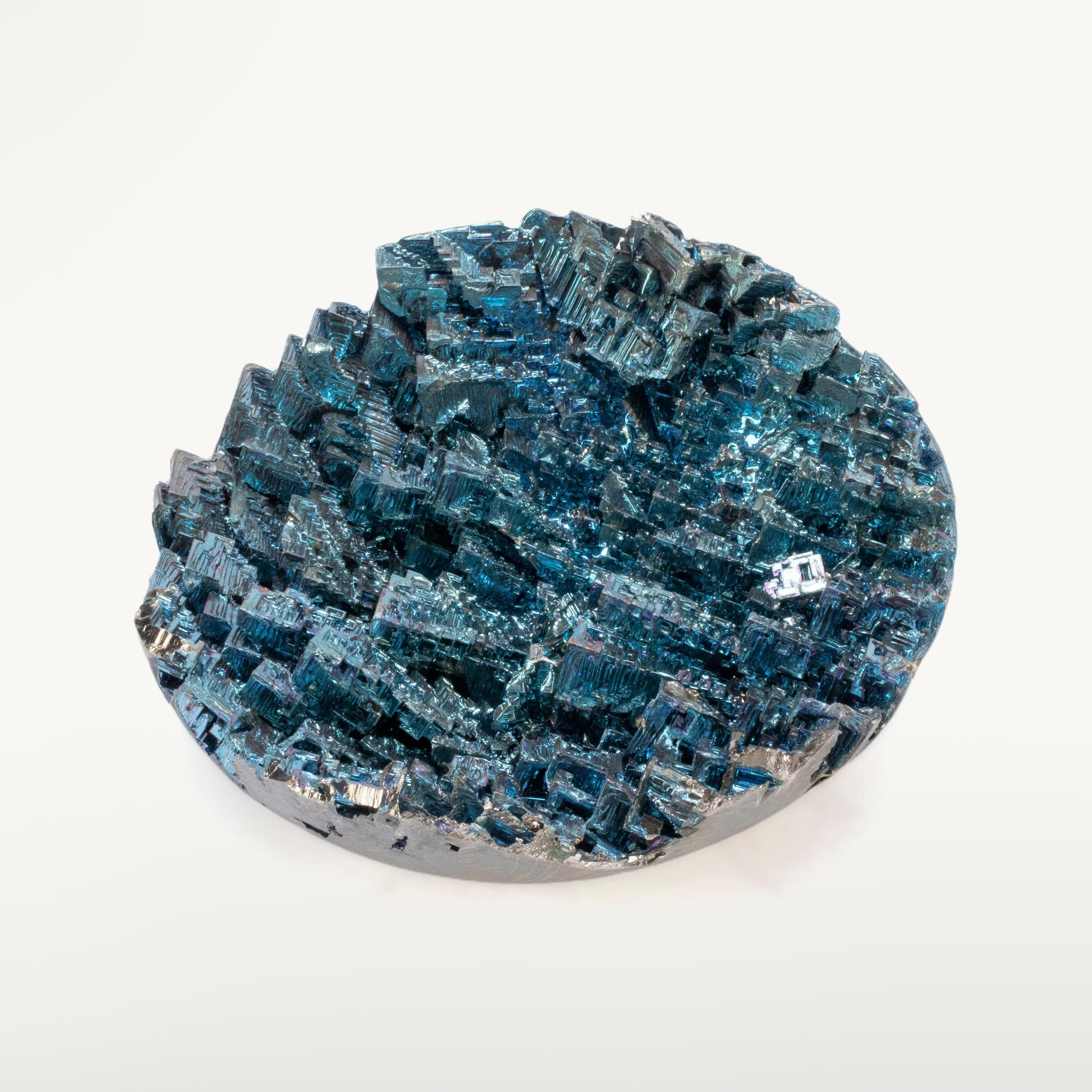The image features a crystal rock set against a plain, entirely white background. The crystal rock, prominently positioned at the center of the photograph, exhibits a circular shape with smooth edges that appear to be silver in color. The majority of the crystal structure is composed of numerous small, square formations stacked upon one another, giving it a rugged and sharp appearance. The interior of the crystal displays a stunning array of blue hues, ranging from navy and light blue to teal and grey-blue, with various sections glistening and reflecting the light, adding a luminous quality to the crystal. The intricate crystal structures and the vibrant color palette dominate the image, making it the sole focus amidst the stark, white backdrop.